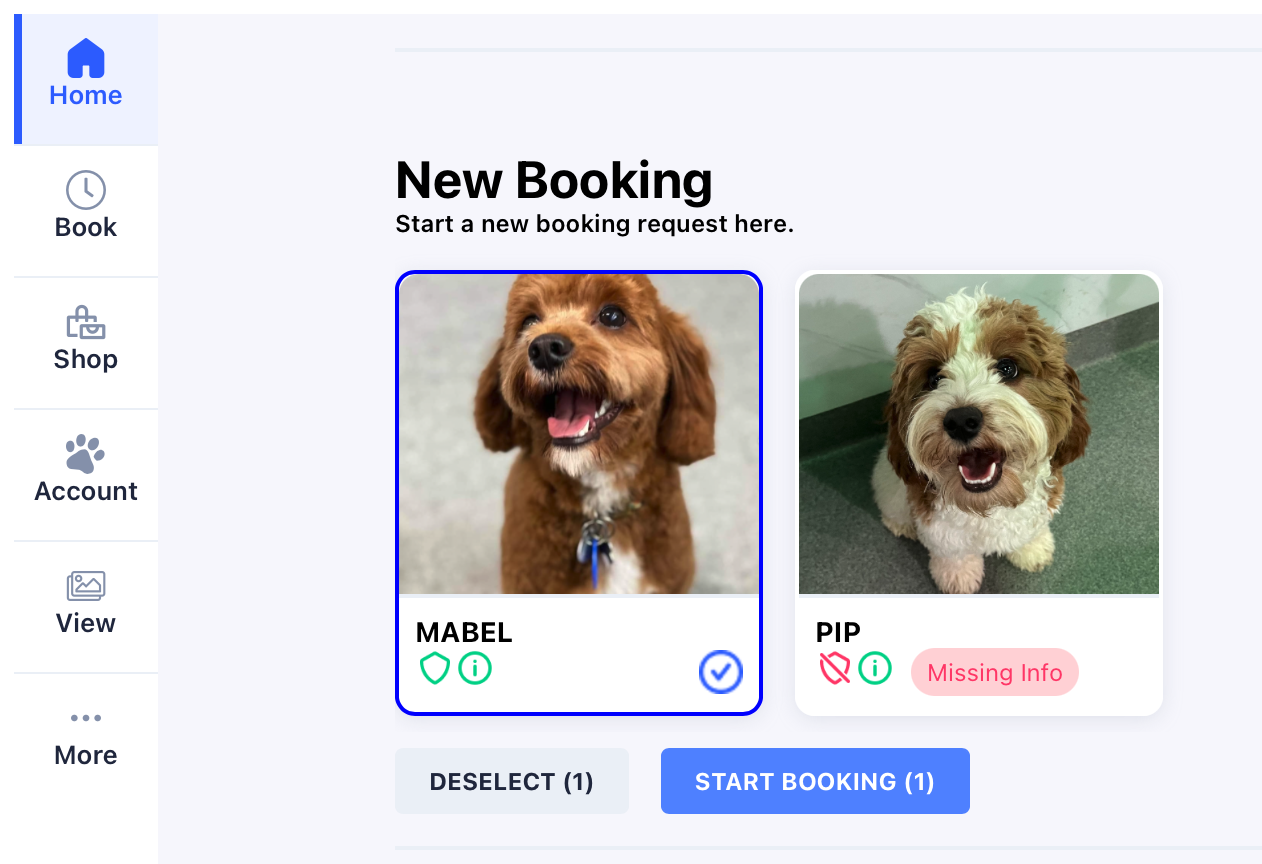The image is a detailed screenshot of a dog booking website. On the left side of the screen are six tabs arranged vertically, labeled as Home, Book, Shop, Account, View, and More. The Home tab appears to be selected, displaying its content on the main screen. At the top center, the main screen shows the title "New Booking" accompanied by the subtext, "Start a New Booking Request here."

In the middle of the screen, there are photos of two small dogs. The dog on the left, named Mabel, is enclosed in a blue selection box, indicating it has been chosen. The dog on the right is named Pip. Below the dogs' photos, there are two buttons: a grey button labeled "Deselect" on the left and a blue button labeled "Start Booking" on the right.